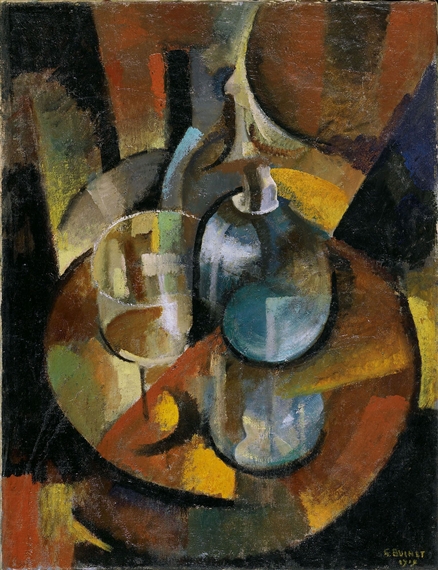This vertical rectangular painting, created in 1919 by Gustave Boucher and titled "Glass and Carafe, Veret et Carafon," is an exemplary piece of cubist artwork. Predominantly rendered in muted earth tones including yellowish-orange, black, brown, gray, with accents of blue, white, and red, the painting employs oil paints to create a textured and fragmented depiction. Central to the composition is an oval-shaped, blue circular object with a reflective base, which is flanked on the left by a partially visible drinking glass with a slightly offset stem. The piece also features various shapes and patterns that suggest elements such as a snail-shaped object in gray and brown and fragmented forms that could represent wine glasses or a tray with dishes. The background is a complex array of irregular shapes and colors, featuring predominantly dark red and black at the top, with additional splashes of yellow and blue towards the bottom. The painting is signed "E. Bulnit 99" in the lower right-hand corner, adding to its historical and artistic significance.